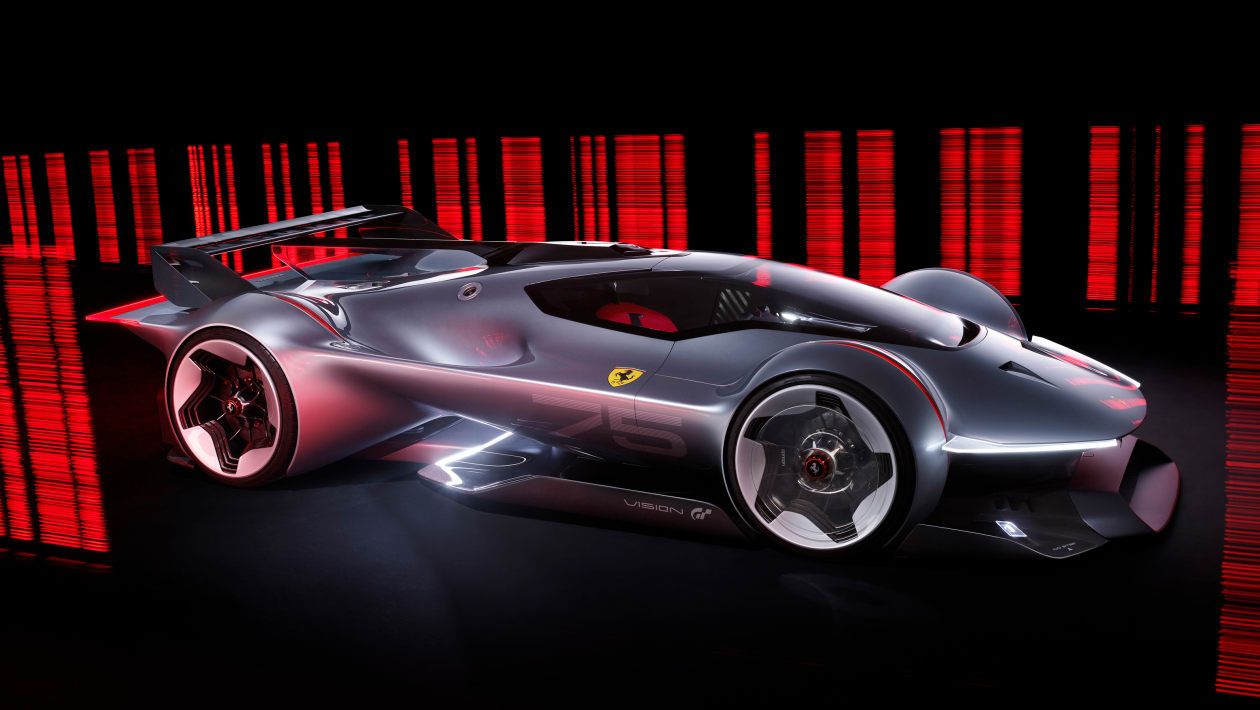In the image, a 3D-rendered, futuristic sports car—or possibly a race car—takes center stage on a dark platform, with a striking red and white striped background that evokes a barcode-like appearance. The vehicle, a gleaming metallic silver, showcases an ultra-streamlined, bullet-shaped design that enhances its aerodynamic profile, suggesting it’s built for speed.

The driver's area is minimalistic, with a single, elongated and small windshield that flows seamlessly into the car’s body. The car appears to be a one-seater, emphasizing its focus on performance. The wheels are particularly noteworthy, with fully encased, shiny silver wheel wells and metallic rims featuring white spoke designs and red caps, giving the vehicle an almost mechanical, AI-generated feel.

Additional design elements, such as the futuristic thin lights positioned at the top, and the absence of traditional doors—suggesting ingress and egress through the top—contribute to its prototype-like appearance. Branding details include the word "Vision" emblazoned on the car, along with a Ferrari logo and the number 75 on its side. The rear of the car features a large carbon fiber spoiler and a unique rack-like structure, reinforcing its high-speed, race-ready characteristics.